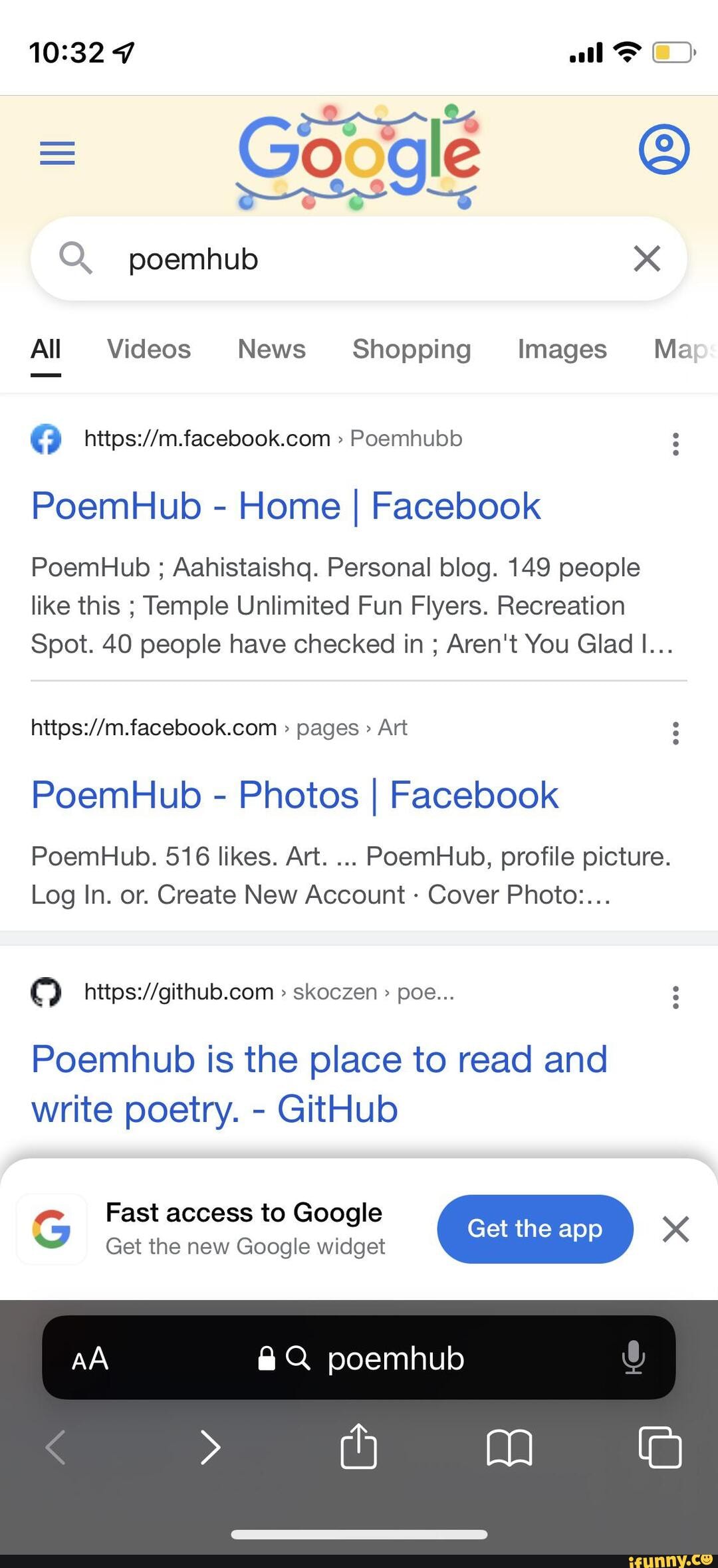**Detailed Caption:**

This image features a screenshot of a Google search conducted on a cell phone. The predominant background color of the interface is white, accented with a dark grey navigation bar at the bottom and a cream-colored Google header at the top.

**Top Section:**
- **Top Left Corner:** Displays the current time as **10:32**.
- **Top Right Corner:** Shows various icons indicating signal strength, Wi-Fi connectivity, and battery power levels.

**Header and Google Banner:**
- The Google banner has a pale cream hue and contains a Google doodle. This particular doodle is the word "Google" displayed in the traditional Google colors, adorned with multicolored fairy lights both above and below the text.
- **Left Side of Banner:** Features a stack of three horizontal lines, representing the menu.
- **Right Side of Banner:** Displays a circular icon with a line drawing of a person, serving as the profile picture.

**Search Bar:**
- **Contents:** Someone has entered the query **"Poem Hub"**.
- **Left:** The search query is preceded by a magnifying glass icon indicating the search function.
- **Right:** An 'X' icon to clear the search bar content.

**Search Results Tabs:**
- Display standard search result categories: **All**, Videos, News, Shopping, Images, Maps, with the **"All"** tab currently selected.
  
**Search Results:**
1. **First Result:** A link to a Facebook page titled "Poem Hub Home on Facebook."
2. **Second Result:** Another link to Facebook content, labeled "Poem Hub Photos Facebook."
3. **Third Result:** A different website, presenting "Poem Hub is the place to read and write poetry" hosted on GitHub.

**Bottom Section:**
- **Google Widget Offer:** A white pop-up bar prompts the user to get a new Google widget.
  - **Left:** Displays the Google "G" symbol.
  - **Center Text:** "Fast access to Google. Get the new Google widget."
  - **Right:** A blue pill-shaped button labeled "Get the app" and an 'X' icon to close the offer.

**Dark Grey Website Bar:**
- **Left Side:** Consists of a smaller 'A' and a larger 'A' for text-size adjustments.
- **Center:** Contains a padlock icon, a search option, and "Poem Hub" written in white.
- **Right Side:** Includes icons for navigation (left and right arrows), sharing, bookmarking, and duplicating tabs.

This descriptive caption meticulously captures all the visual elements and details presented in the screenshot.